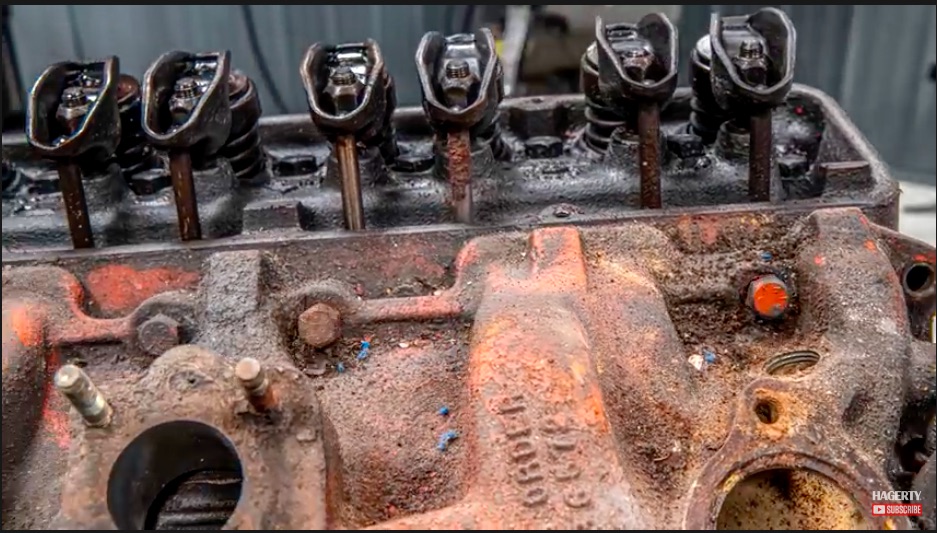This photorealistic close-up image showcases the aged and intricate details of a rusted engine, likely from a car, split into two distinct sections. The bottom half, predominantly a deep rust color, highlights the extensive wear and tear, featuring three bolts securely fastened into the side, and faint text etched into the metal reading "ORDH6672." Two silver cylinders can be seen protruding from this area, suggesting mechanical complexity. The top half contrasts with a darker gunmetal gray, displaying five upright components resembling flower-like valves, indicating parts of the engine in better condition, though still aged with oil stains. In the blurred background, a workshop setting provides context, reinforcing the engine’s utilitarian past. A watermark in the lower right corner reads "Hagerty," accompanied by the YouTube logo and the word "Subscribe," adding a modern layer of branding to this image of vintage machinery.